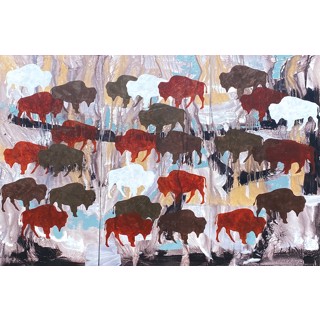This image showcases a vibrant watercolor painting split into three canvas pieces, resembling an abstract art piece. It features numerous silhouettes of bison or buffalo, depicted in various colors such as white, red, brown, gray, and dark green. The buffalo appear to be grazing and are oriented in different directions—some facing right and others facing left. Their movements form lines and circles, creating a sense of dynamic motion. The background is a striking mix of smeared and blended colors, including shades of blue, white, purple, beige, orange, pink, and black, resembling a tie-dye pattern. The overall composition is both colorful and abstract, with the multitude of buffalo emphasized through a stamping technique, giving the impression that they are part of a boundless, lively herd against a vividly textured backdrop.